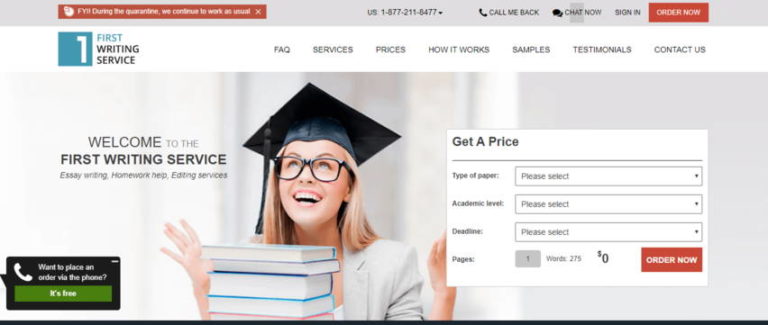**Descriptive Caption:**

This screenshot captures a writing service website with a user-friendly interface and various useful features. At the top, there's a gray bar housing an orange "FYI" button. The main functional area beneath the gray bar includes multiple interactive elements:

- On the far right, an orange button reads "Order Now," accompanied by a blue box displaying the number "1."
- Below these are options for first-time writing a VAT, as well as links to the FAQ, Services, Prices, How It Works, Samples, Testimonials, and Contact Us sections.

Prominently displayed is an image of a woman wearing a graduation hat and glasses. She gazes upwards, with her hands raised near her shoulders, and a stack of books is positioned in front of her. To the left of her image, inviting text reads: "Welcome to the First Writing Service," followed by "Easy Essay Writing," "Homework Help," and "Services."

In the bottom-left corner, there is a phone icon next to a black speech bubble that offers the option: "Want to place an order via the phone? It's free." A green button accompanies this prompt.

To the right of the woman's image, there are fields to customize an order. These include:

- "To make a VAT, type a paper," followed by drop-down menus for "Academic Level," "Deadline," and a box to enter the number of words.
- Default selections show "Papers: 1," "Words: 275," and a price of "$0."

An orange "Order Now" button is also included here for finalizing the order.